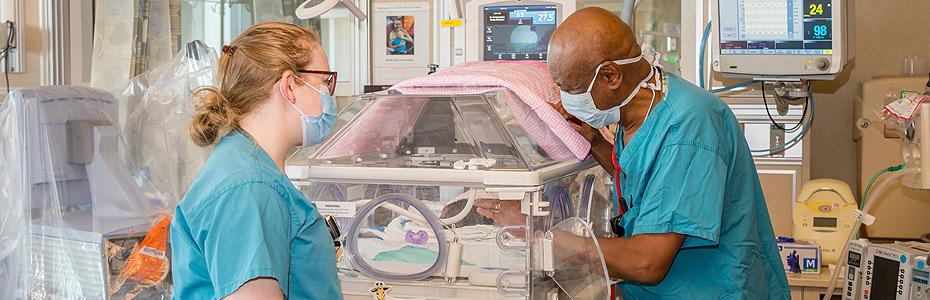In a bright, modern NICU infant critical care unit, the scene captures two healthcare professionals deeply engrossed in their tasks. The central focus is an incubator, a transparent plastic case with sterile inlets, inside which lies a baby with dark hair, partially visible. An African-American man in surgical scrubs and a blue face mask, possibly a doctor, is reaching through the side hand holes to touch the infant's head, his stethoscope hanging around his neck. Opposite him, a white woman in scrubs and glasses, also wearing a mask, observes attentively—potentially another doctor or a nurse. They are surrounded by various medical monitors and machines, including a heartbeat and blood pressure monitor, all indicating a state-of-the-art medical setting. Additional details include a pink blanket draped over the incubator and a pacifier inside, alongside a box of gloves and other essential medical equipment scattered in the background.